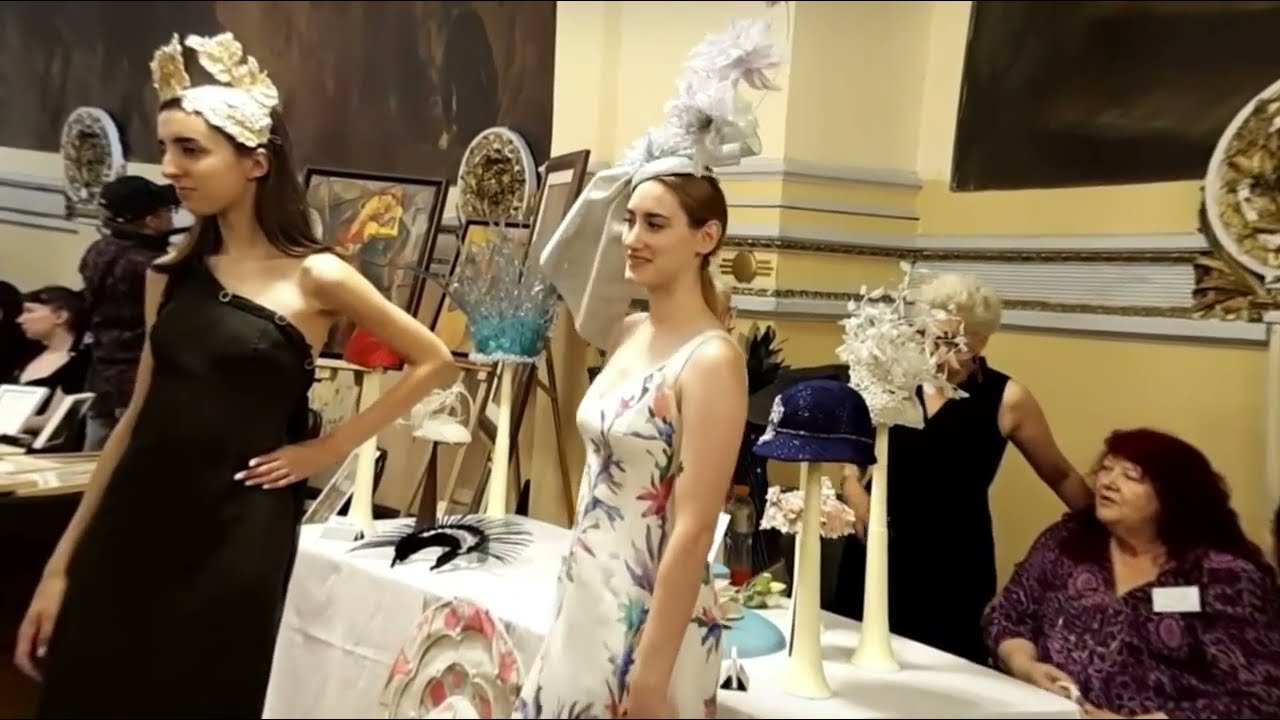In an elegantly decorated room with yellow walls, possibly an art gallery or an exhibition hall, two young women stand facing to the left, showcasing extravagant hat designs. The woman closest to the camera is dressed in a stylish black, one-shoulder dress, with her bare left shoulder visible. She wears an intricate white hat resembling paper mache. Standing just behind her, slightly higher, is another woman sporting a large, bowl-like white hat and a floral print dress. Both women exude sophistication, fitting the theme of what appears to be a hat fashion show.

Behind them, a long table is set up with various elaborately designed hats on display, suggesting that the event is being judged. Seated at this table are several women, perhaps the judges, indicating a formal evaluation or showcase of the hats. To the left, an assortment of pictures, mirrors, and additional artwork adorns the walls, enhancing the artistic ambiance of the space. The entire scene combines elements of fashion and art, emphasizing the detailed craftsmanship of the headpieces and the elegant presentation of the event.